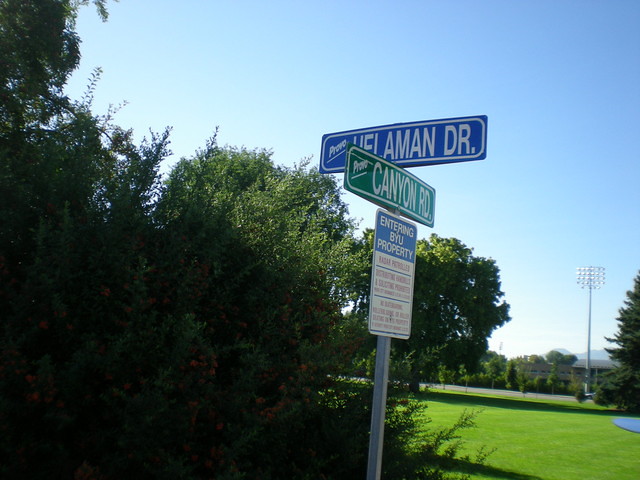In this detailed color photograph, the central focus is a grey pole with three attached signs, positioned against a backdrop that features both natural and man-made elements. The topmost sign, which we see at an angle, reveals a blue background with partially readable white text that likely says "Amon Drive." Directly below, a green sign reads "Canyon Road" in white writing and is oriented diagonally. The third sign at the bottom also has a blue upper section with unreadable white text and a white lower section with small red text. 

Surrounding the pole, the left side of the image is dominated by a large green tree extending its branches towards the center, hinting at a wooded area behind. In contrast, the right side includes a light green grassy field, smaller trees, an electricity pole in the distant background, and what appears to be a far-off building. The sky above transitions from white at the horizon to a light blue towards the top of the frame. Near the bottom left corner, part of the image is entirely black, creating a stark contrast to the vibrant colors of the signs and natural surroundings.